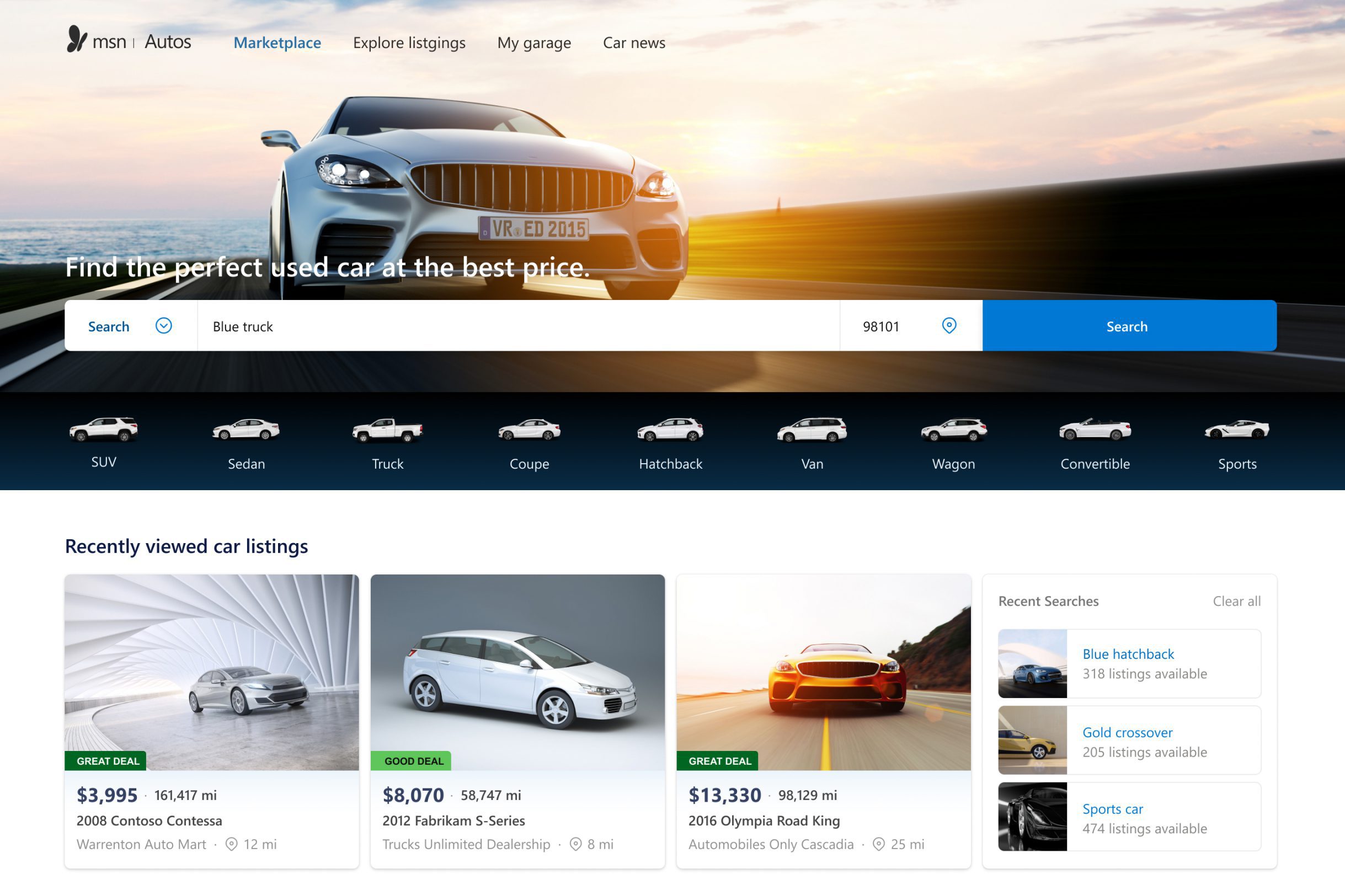The image showcases a detailed layout of a car marketplace website interface. At the top, on the left, there is a black silhouette of a butterfly icon, followed by the text "MSN Autos." Below that, in blue text, there are sections labeled "Marketplace," "Explore Listings," "My Garage," and "Car News." The background is a beautiful sunset over the ocean to the left, with a dark grassy hill to the right. On the road, a white sports car is driving, adding to the scene's dynamic feel.

Prominently displayed in white text is the tagline, "Find the perfect used car at the best price." Below this is a long white rectangle featuring a search bar with the text "Blue Truck" pre-filled. To the right of the search bar, a blue "Search" button is present. Underneath, there are various category images representing different car types: SUV, Sedan, Truck, Coupe, Hatchback, Van, Wagon, Convertible, and Sports.

Additionally, the interface shows a section for recently viewed car listings, which includes a 2008 Contessa priced at $3,995, a 2012 Fabrikam S-Series priced at $8,070, and a 2016 Olympia Road King priced at $13,330. At the bottom, the recent searches section displays entries such as "Blue Hatchback," "Gold Crossover," and "Sports Car," all highlighted in blue. The comprehensive layout is user-friendly and visually appealing, providing a streamlined car shopping experience.